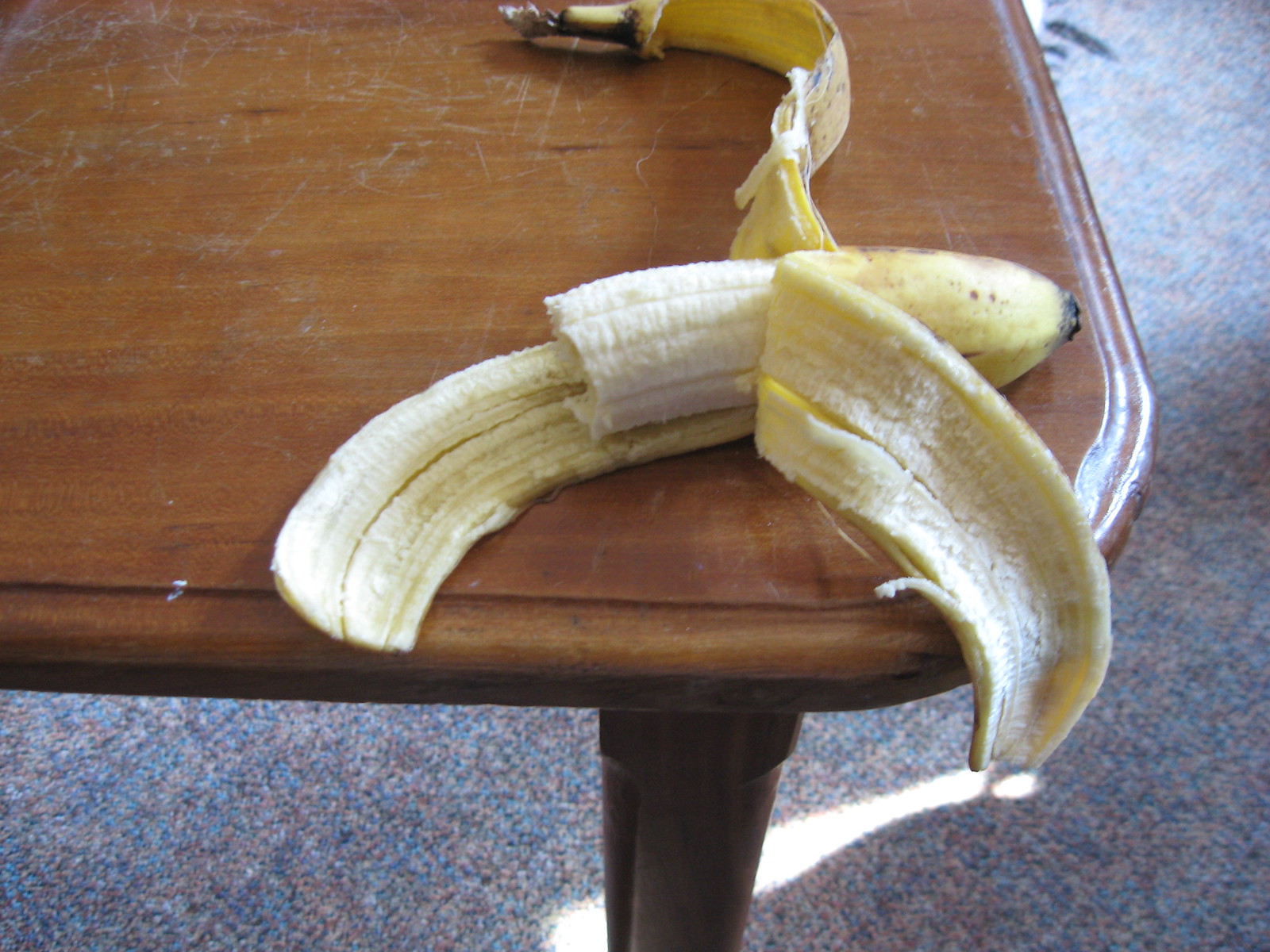A vivid color photograph depicts a partially eaten banana resting on a worn wooden coffee table. The ripe yellow banana, half-consumed, sits propped on one-third of its peeled skin, while the remaining two peels drape across the table’s surface. The table, showing signs of wear and tear with noticeable scuff marks, stands atop a carpeted floor featuring a textured blend of greenish-blue and beige fibers. Sunlight streams through a window off to the right, casting gentle light onto the carpet and enhancing the cozy ambiance of the scene. The banana’s exposed portion clearly reveals bite marks, indicative of someone having eaten it directly. No people, hands, or utensils are in view, leaving the focus solely on the simple yet intimate setting.